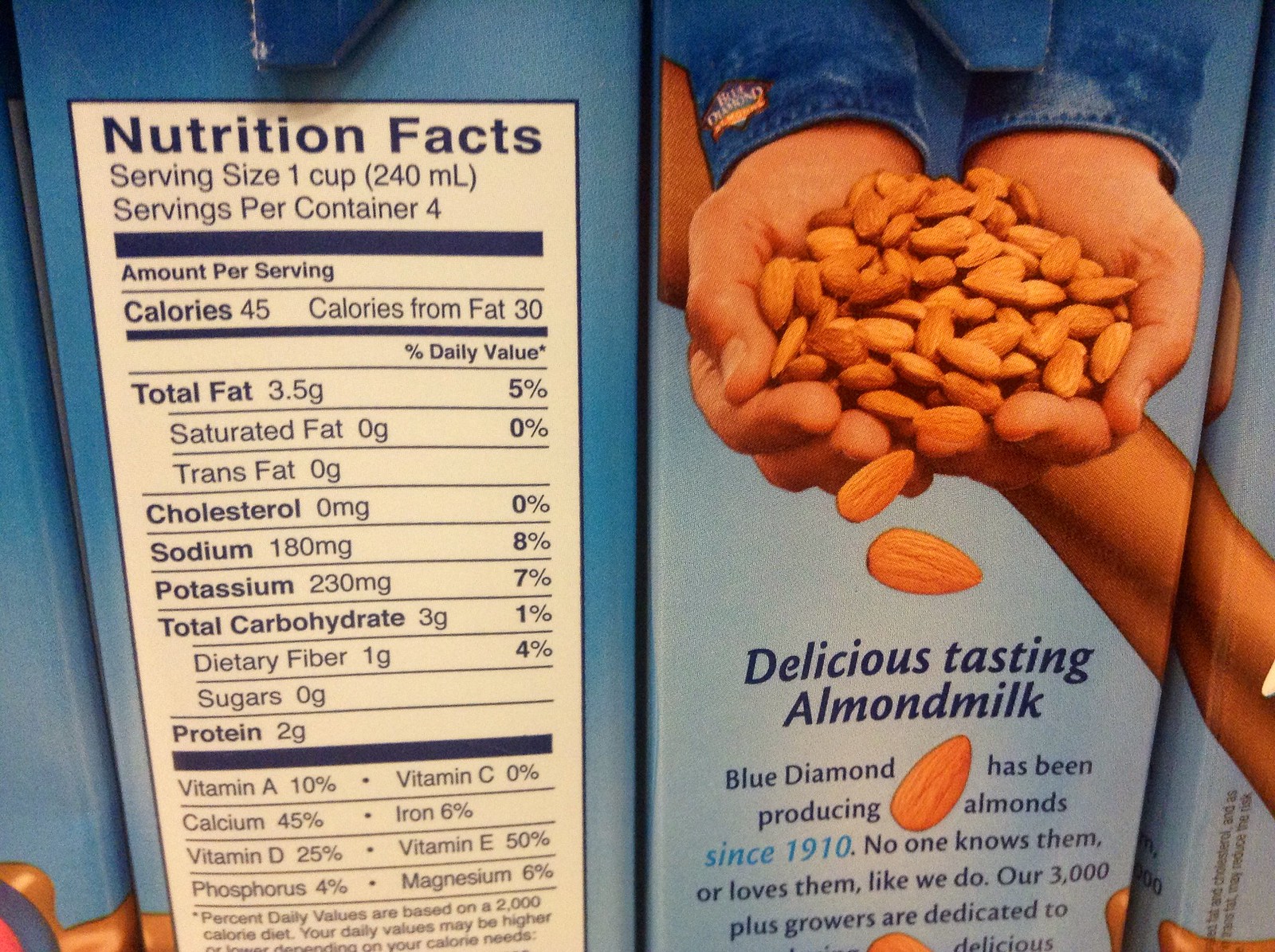The image is a color photograph showcasing a close-up row of almond milk cartons blending seamlessly into each other. Each carton has a distinctive design featuring two main panels. One panel, set against a light blue background with a dark blue overlay, prominently displays the Nutrition Facts. This section, framed by a cream-colored box, details vital nutritional information including serving size (1 cup), servings per container (4), calories (45), calories from fat (30), total fat, saturated fat, trans fat, cholesterol, sodium, potassium, total carbohydrate, dietary fiber, sugars, protein, vitamin A, calcium, vitamin D, phosphorus, vitamin C, iron, vitamin E, magnesium, and the percent daily values based on a 2000 calorie diet.

The other panel is more visually engaging, featuring a photograph of a pair of fair-skinned hands, clad in a denim shirt, gently cupping a pile of almonds, with some almonds cascading down. This panel includes a slogan that reads, "Delicious tasting almond milk. Blue Diamond has been producing almonds since 1910. No one knows them or loves them like we do." Further details are obscure due to the image being cut off. The overall aesthetic of the packaging merges practical nutritional data with engaging imagery, underscoring Blue Diamond's rich heritage and dedication. In the background, additional cartons replicate the design, creating a continuous visual flow.